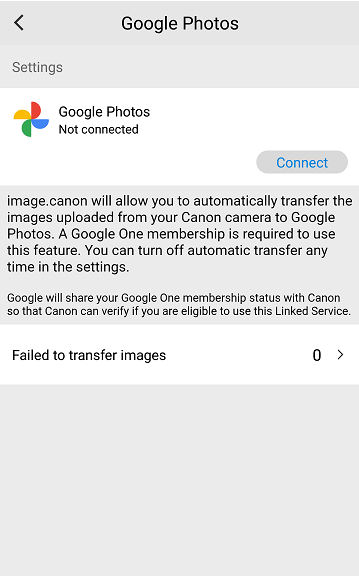This image appears to be a screenshot of a smartphone displaying settings related to the Google Photos app. At the top of the screen is a grey navigation bar with a black back arrow on the left, and the text "Google Photos" prominently centered in black. Below this, there is a section labeled "Settings" on the left side. 

A white background hosts a status message indicating that "Google Photos is not connected," accompanied by the Google Photos icon, which features a windmill with yellow, red, blue, and green blades. To the right of this message is a grey button with the text "Connect" in blue font.

Further down, another grey rectangle contains a black text explanation: "image.canon will allow you to automatically transfer the images uploaded from your Canon camera to Google Photos. A Google One membership is required to use this feature. You can turn off automatic transfer any time in the settings. Google will show your Google One membership status with Canon so that Canon can verify if you're eligible to use this linked service."

Beneath this text is a white rectangle displaying another message: "Failed to transfer images" with a count of zero, followed by a small arrow pointing to the right.

Finally, near the bottom, there is another grey rectangle consistent in color with the earlier elements on the screen. This detailed context suggests this screenshot may indeed be from an interface related to linking a Canon camera with Google Photos, rather than a typical Google Photos screen.